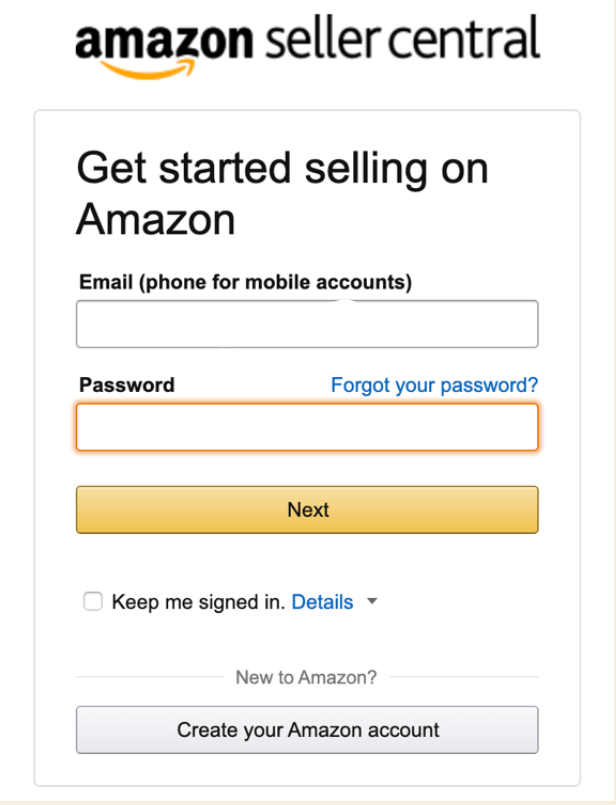This image appears to be a screenshot from the Amazon Seller Central application. At the very top, there is a prominent Amazon logo featuring the iconic yellow smile. Adjacent to the logo, the text "Seller Central" can be seen. Below this header, there is a box that guides users to start the registration process for selling on Amazon. The heading within the box states, "Get started selling on Amazon" in bold text.

Immediately below the heading, there is a field labeled "Email (phone for mobile accounts)" with an input textbox for users to enter their email or phone number. Following this, another field labeled "Password" is displayed, accompanied by a tooltip in blue text: "Forgot your password?" There is also an input textbox for users to enter their password, highlighted with an orange border.

Below these input fields, a yellow button labeled "Next" is prominently displayed. Further down, there is an unchecked checkbox option labeled "Keep me signed in," next to which is a link "Details" in blue font, alongside a down arrow indicating a drop-down menu option. At the very bottom of the box, there is text indicating, "New to Amazon?" followed by a light gray button that prompts users to "Create your Amazon account."